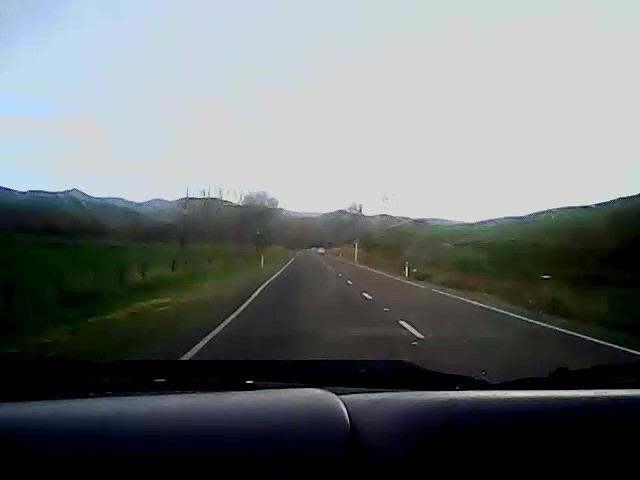A photograph captures the ambiguous view from a vehicle driving on a highway. The perspective suggests we could be looking through either the front or rear windshield because of the visible hood area and a faint reflection hinting at windshield wipers. The image quality is unclear, making it challenging to determine the exact driving direction. In the distance, indistinct cars navigate the road, bordered by hilltops and scrubland. The asphalt highway features lane markers, but it's indeterminable whether the observed cars are approaching or receding. The scene unfolds under an overcast sky, adding to the photo's enigmatic nature.